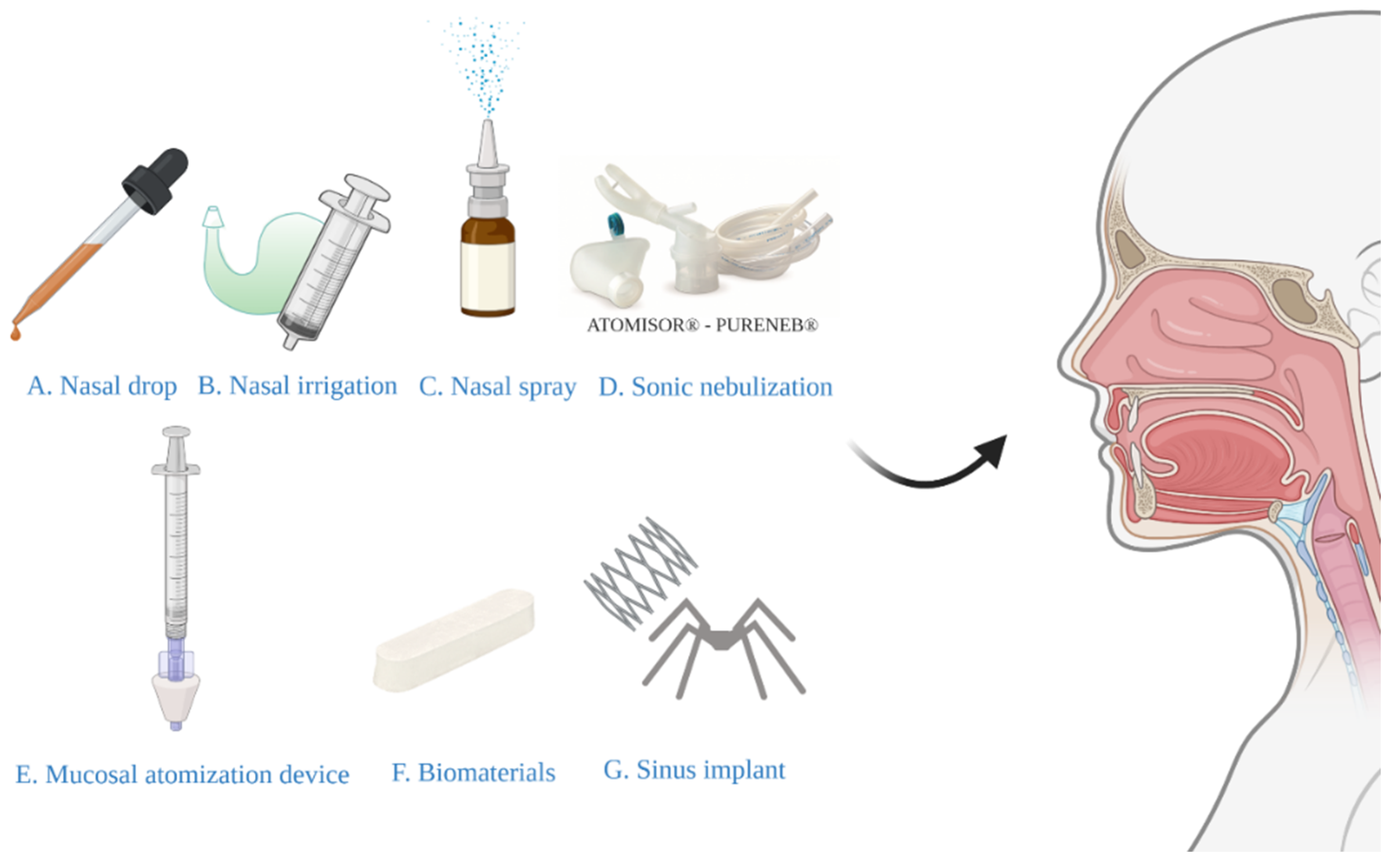The image is a detailed medical diagram showcasing various sinus treatment devices labeled A through G, positioned alongside a human head illustration depicting the anatomy of the nose, mouth, throat, and trachea. 

- **A: Nasal Drop** - Depicted in blue font, this item is an eyedropper containing orange or brown liquid, with a black rubber tip.
- **B: Nasal Irrigation** - Represented by a syringe-like device with a green design in the background, resembling an elephant trunk. This device is used to blow solutions up the nose.
- **C: Nasal Spray** - Shown as a brown bottle with a white top, emitting blue droplets to indicate its spraying action.
- **D: Sonic Nebulization** - Illustrated as complex equipment including an atomizer with one part resembling an inhaler and another with two prongs. 
- **E: Mucosal Atomization Device** - A syringe-like apparatus with an upside-down white triangle at the end meant for delivering medication without a needle.
- **F: Biomaterials** - Illustrated as a long, skinny rectangle resembling a white eraser or a curved-end brick.
- **G: Sinus Implant** - Visually compared to a creepy metal spider and a device with sharp teeth or metal springs, indicating its use inside the sinus cavity.

This array of devices is specifically designed to address various conditions and treatments related to nasal and sinus issues.